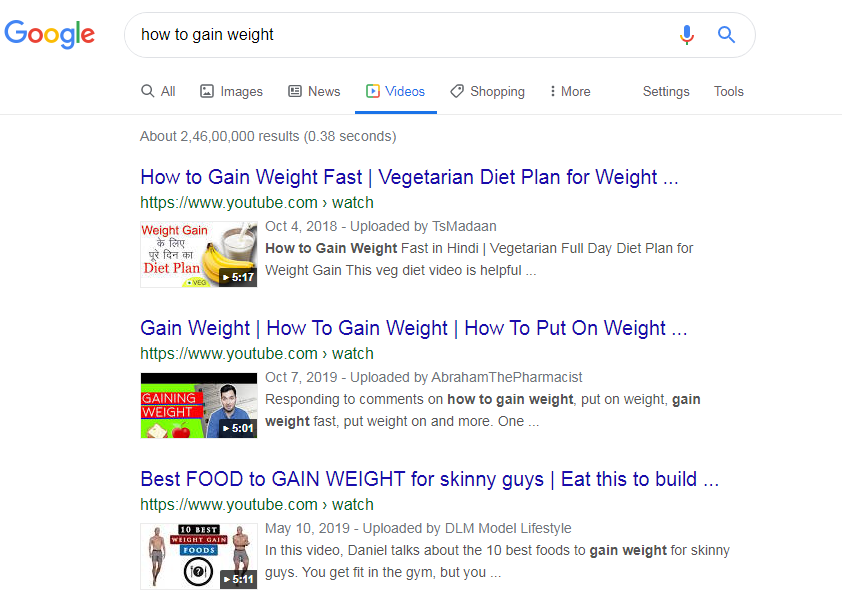The image showcases a Google search results page. On the top left, there is the recognizable Google logo featuring the letters "G" in blue, "O" in red, "O" in yellow, "G" in blue, "L" in green, and "E" in red. In the search bar, the query "how to gain weight" has been entered. 

Below the search bar, there are tabs for different types of results: "All," "Images," "News," "Videos," "Shopping," and a menu represented by three vertical dots for additional options like "More settings" and "Tools." The "Videos" tab is highlighted in blue.

The search returns approximately 2,446,000 results in 0.38 seconds. The first result is a YouTube video titled "How to Gain Weight Fast Vegetarian Diet Plan for Weight" from youtube.com. The second result is titled "Gain Weight: How to Gain Weight, How to Put on Weight," also from youtube.com. The third result is "Best Food to Gain Weight for Skinny Guys: Eat This to Build," again from youtube.com. All titles are displayed in blue, and each YouTube link is shown in green beside a green "Watch" button.

Under each video title, there is additional information in gray text, specifying the upload date: the first video is from 2018, the second from 2019, and the third also from 2019.